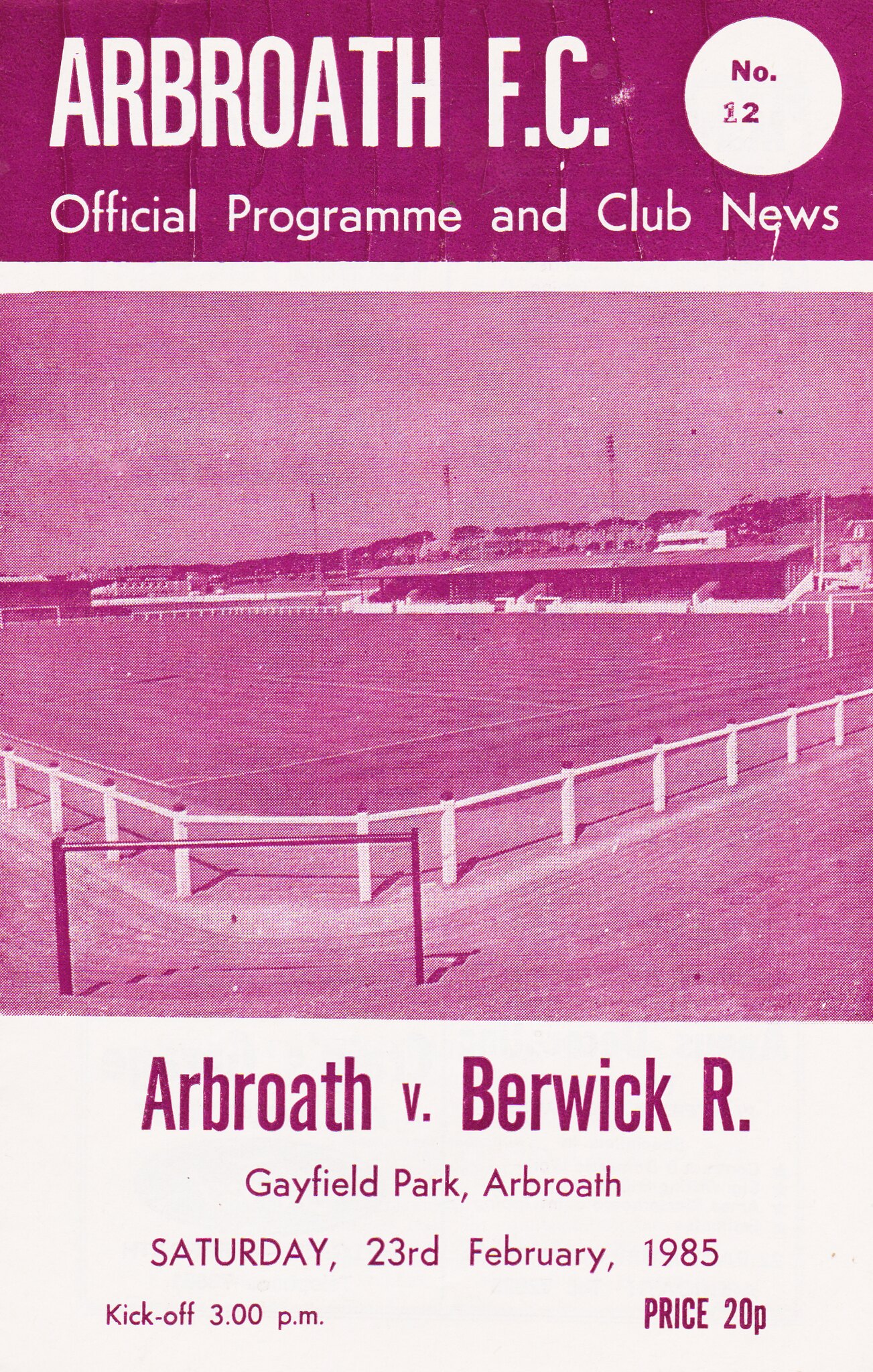The image is likely a cover for a sports program or magazine, prominently featuring a purplish-pink background at the top. It is divided into three panels. At the very top, a pink rectangle displays the words "Our Broth FC" in white. Adjacent to it, within a white circle, the number "2" is inscribed. Below, the text "Official Program and Club News" is printed in white letters. 

Further down, separating the sections, there is a broad white space, under which a purple square captures the viewers' attention. This square contains an image that resembles a soccer or football field, encircled by a white fence. Below this image, the text "Arbroath versus Berwick" is printed in purple letters. Additional details include the match location and timing: "Gayfield Park Arbroath, Saturday 23rd February 1985, Kickoff 3 p.m." Finally, the price is stated as "20p."

The background maintains a consistent purplish-pink hue, enhancing the vintage look of the cover.